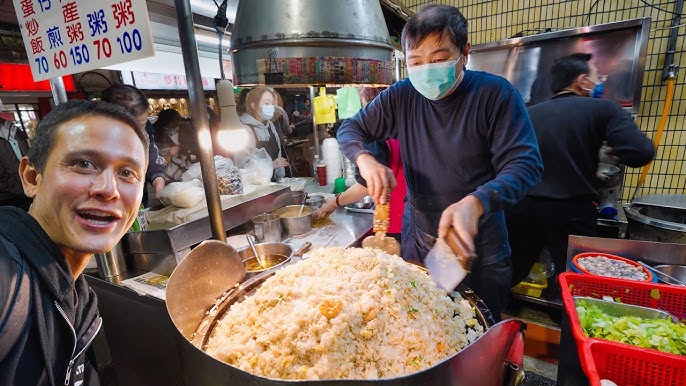This landscape photograph captures a vibrant, bustling scene at an Asian street food market. The central focus at the bottom of the image is a plate of food. Dominating the center is an Asian man in a long-sleeve blue shirt, wearing a mask, and mixing a massive bowl or vat of food that resembles cornmeal using tools in his hands. 

To the left of this man, a second man in a black shirt poses for the camera, smiling broadly with his mouth open, seemingly taking a selfie. Above his head, a white sign adorned with red and blue text in Japanese letters and numbers provides some details, possibly pricing, related to the stall. 

The backdrop reveals a detailed kitchen setup, complete with pots, bowls, shelves, and various cooking utensils, contributing to the busy market atmosphere. In the lower right-hand corner, red Tupperware containing what appears to be onions and lettuce is visible. Additional people can be seen in the background, either working or as customers, further highlighting the lively nature of the street food fair.